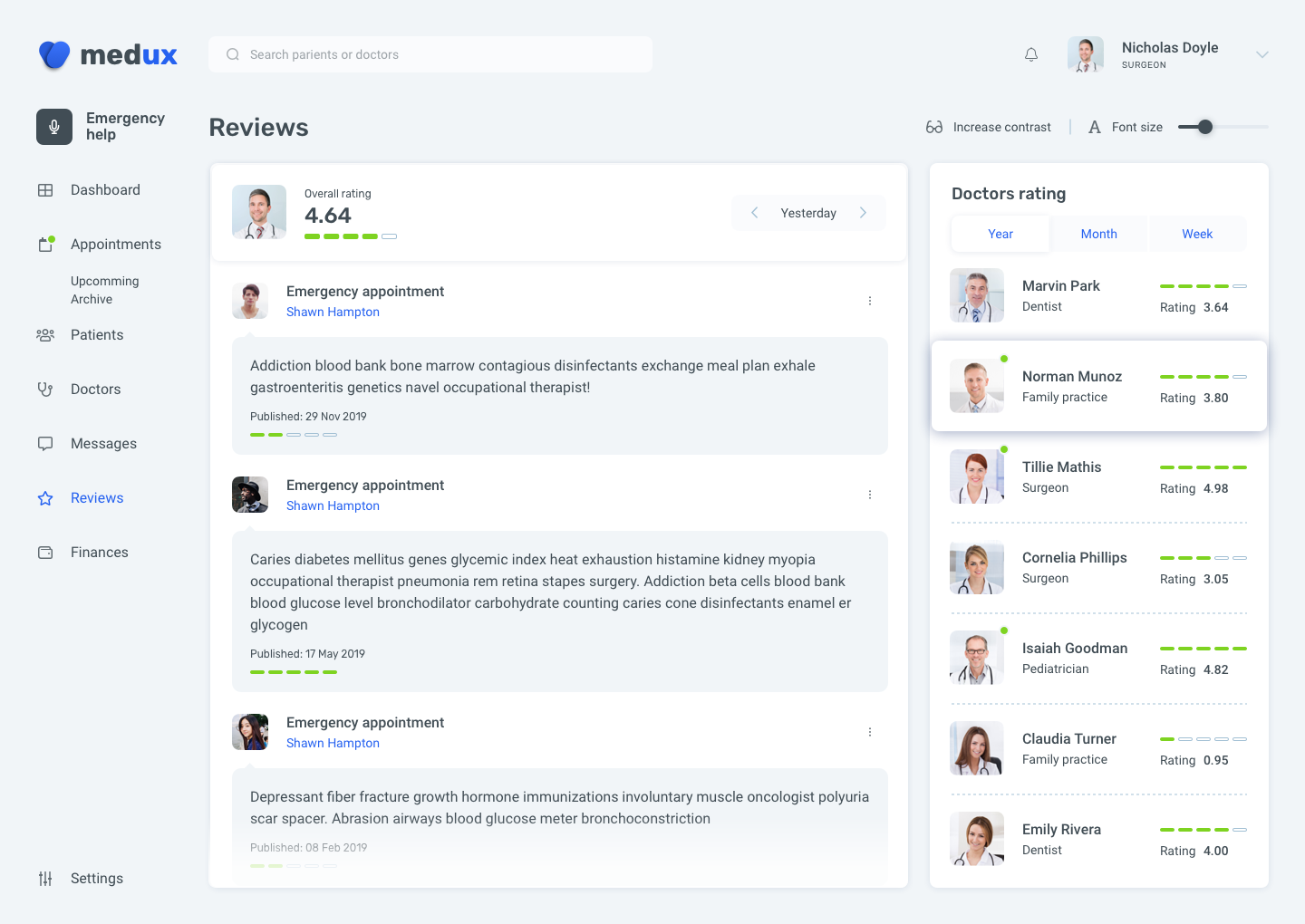**Detailed Caption for the Descriptive Image:**

The web page features a dark grey background, with a clean and professional layout. In the top left corner, there are two lines in dark blue. Across on the right-hand side, the words "med ux" are displayed, with "med" in black and "ux" in dark blue.

Beneath these elements, there is a search bar. The search icon, represented by a grey magnifying glass, sits inside the bar, and the placeholder text reads "Search patients or doctors."

To the right of the search bar, there's a prominent dark blue square. Inside the square is a white microphone icon, accompanied by the text "Emergency Help" in bold dark blue lettering.

On the right-hand side of the page, there's a section dedicated to reviews. This section features a doctor with short black and grey hair, wearing a white coat, red tie, and black stethoscope around his neck. His overall rating is prominently displayed in black text, with a bold "4.64" beneath it. There are four green rectangles and one white rectangle indicating varying levels of ratings.

Within the reviews section, there are also individual reviews. One review features a person with light skin, brown hair, and a white shirt, listed for an emergency appointment named Sean Hamilton (with his name clickable in blue). His review lists a series of medical terms and conditions he is associated with, such as "addiction," "blood bank," and "bone marrow," and it mentions his review was published on November 29, 2019, with a rating of two out of five green bars.

Another review section shows an African American individual wearing a grey dress hat, grey tuxedo, grey tie, and a white undershirt. His review, for an emergency appointment, includes various medical terms like "caries," "diabetes," and "glycemic index." His review was published on May 17, 2019, with a perfect rating of five out of five green bars.

A third review highlights an Asian female with shoulder-length brown hair and a black shirt. Her content includes terms such as "depressive fiber fracture" and "growth hormone." Her review also lists multiple medical terms and conditions.

On the left side of the webpage, a sidebar menu includes options: Dashboard, Appointments, Upcoming, Archive, Patients, Doctors, Messages, and the currently selected Reviews, which is highlighted with a blue star. Each section, except Reviews, is grey. Below this menu, a folder labeled "Finances" and a section named "Settings" with multiple lines and dots end the sidebar.

Overall, the interface is user-friendly and provides detailed information prominently and accessibly, aiding in effective navigation and review of medical professionals and appointments.